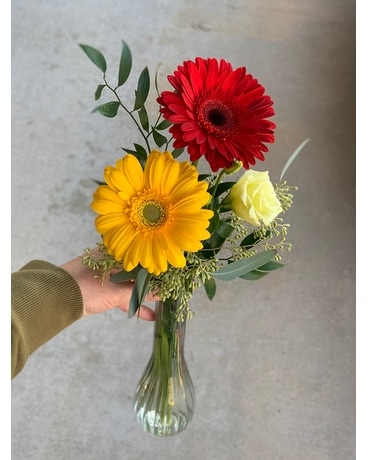In this detailed image, a Caucasian person, wearing a long-sleeved greenish sweater, is holding a glass vase in midair against a bluish-purple background. The vase, filled with water, contains an arrangement of vibrant flowers. Prominently featured are three main blooms: a yellow sunflower with a characteristic crown adorned with lighter green parts at its center, a dark red sunflower with a distinctive black ring at its core, and a delicate white rose. Additionally, smaller green stems and leafy branches accentuate the main flowers. These additional elements, akin to baby's breath, provide a fuller look to the floral ensemble. The hand holding the vase is outstretched, emphasizing the entire floral arrangement as the focal point.